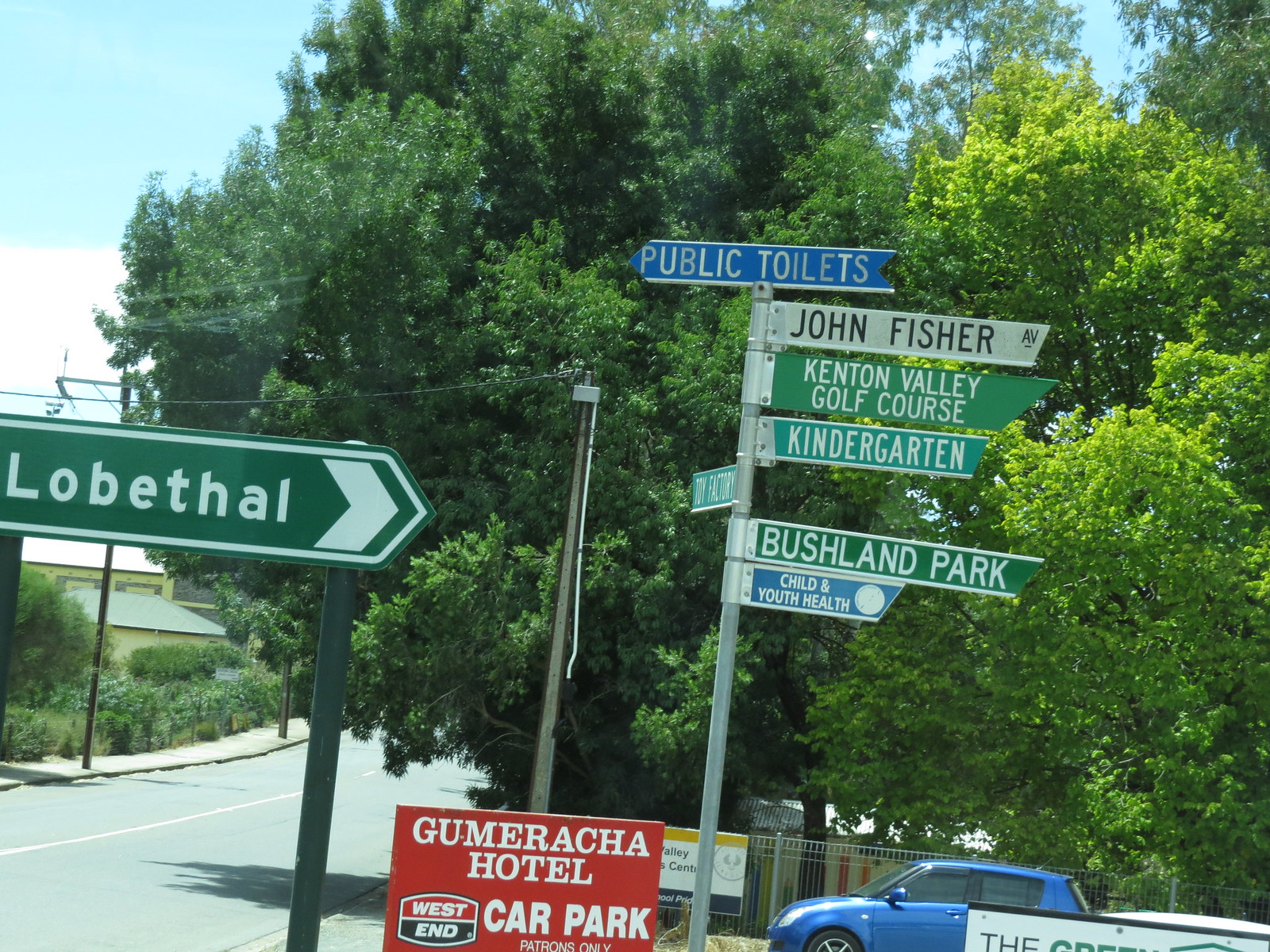In the bright and sunny scene, a busy street sign post stands prominently against a clear blue sky dotted with white clouds. The sign post features multiple directional signs that branch out in various directions. At the top, a blue sign indicates "Public Toilets," followed by a light green sign for "John Fisher Avenue." Below it, a darker green sign points towards the "Kenton Valley Golf Course," and another sign notes the location of a "Kindergarten." Further down, a green sign points to "Bushland Park," and below it, a light blue sign appears to denote "Child and Youth Health." Additionally, a green sign for "Lobethal" points directly towards the sign post, while a red sign beneath it directs towards the "Gumeracha Hotel, West End Car Park." A small blue car is parked next to a fence under a large tree, adding to the rural and tranquil atmosphere. The street to the left is empty, surrounded by more big trees, contributing to the serene, sparsely populated environment.